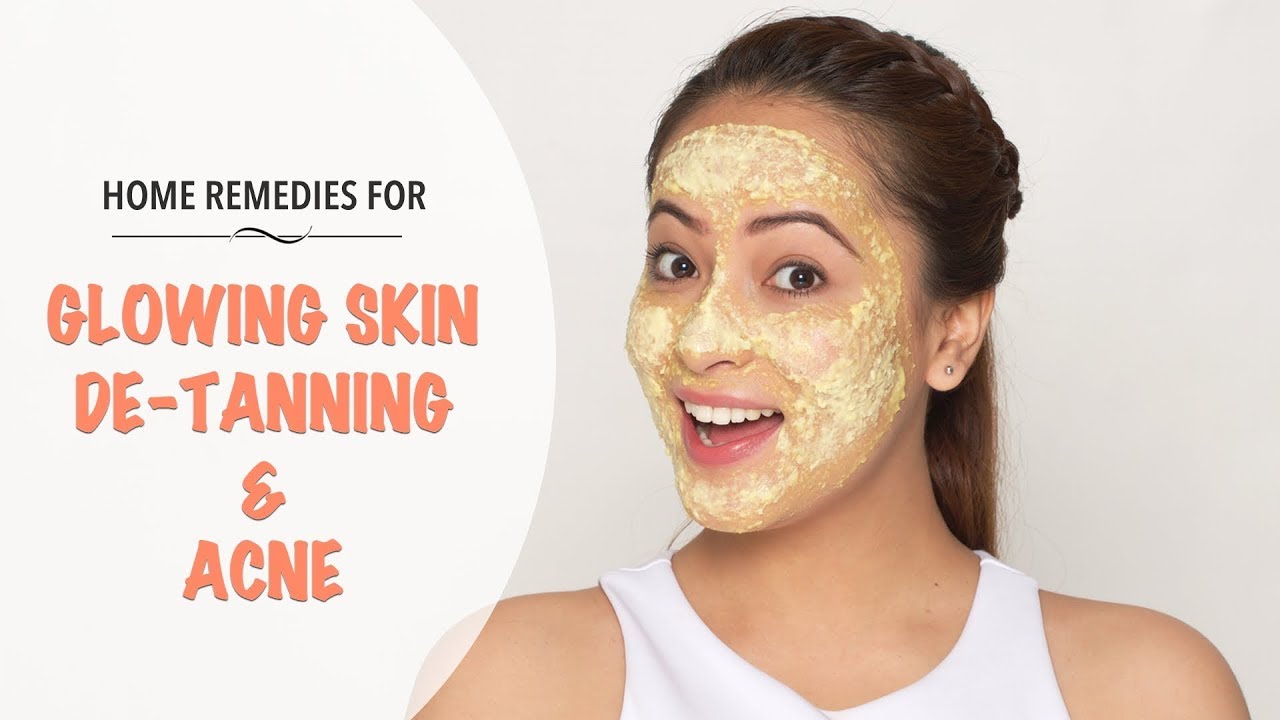The image showcases a web page dedicated to home remedies for glowing skin, de-tanning, and acne, displayed within a white circle on the left side, featuring black and peach-colored text. On the right side, a pretty Caucasian woman, smiling with her wide, proportionate teeth, and brown, arched eyebrows, is captured looking directly at the camera. She has her brown hair pulled back, wears tiny stud earrings, and a sleeveless tank top. The woman, adorned with a facial mask covering her face from her forehead to her chin, is demonstrating how to apply these homemade skincare treatments. The overall composition highlights effective skincare solutions with a personal, relatable touch.